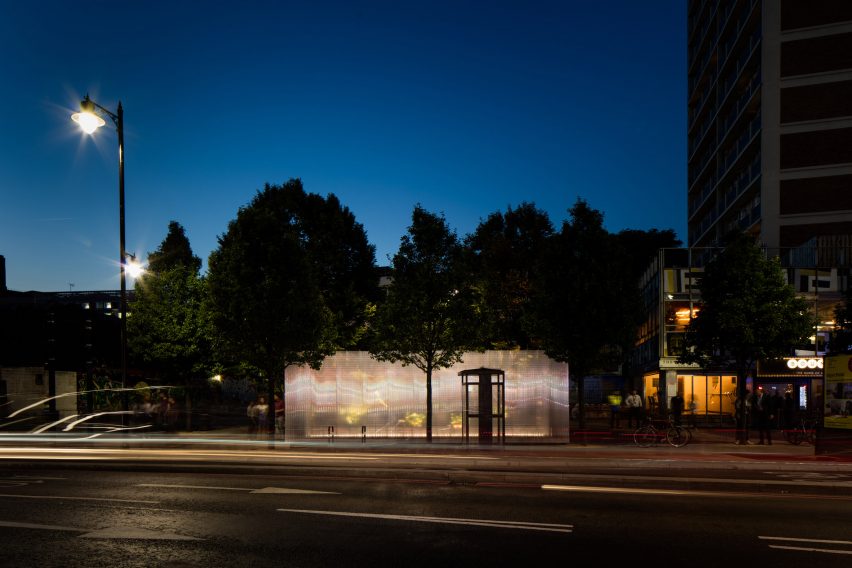This detailed night-time photograph captures an urban scene just as twilight gives way to darkness. Dominating the left side of the image is a tall, illuminated street lamp that casts light onto an empty bus stop with semi-transparent panels and subtle overhead protection benches. The bus stop blends seamlessly into the urban landscape, adding a touch of quiet elegance. In the background, silhouettes of trees and streaks of light from passing vehicles are captured in time-lapse, adding dynamic elements to the stillness. On the far right stands a high-rise building with a dark facade, possibly a hotel, accompanied by a smaller building with lit windows below, hinting at interior activity. The foreground features a black asphalt road marked with white stripes and arrows, indicating a functional, yet aesthetically pleasing urban infrastructure. Overall, the image encapsulates a serene moment in a city night, characterized by its detailed interplay of light and shadow.